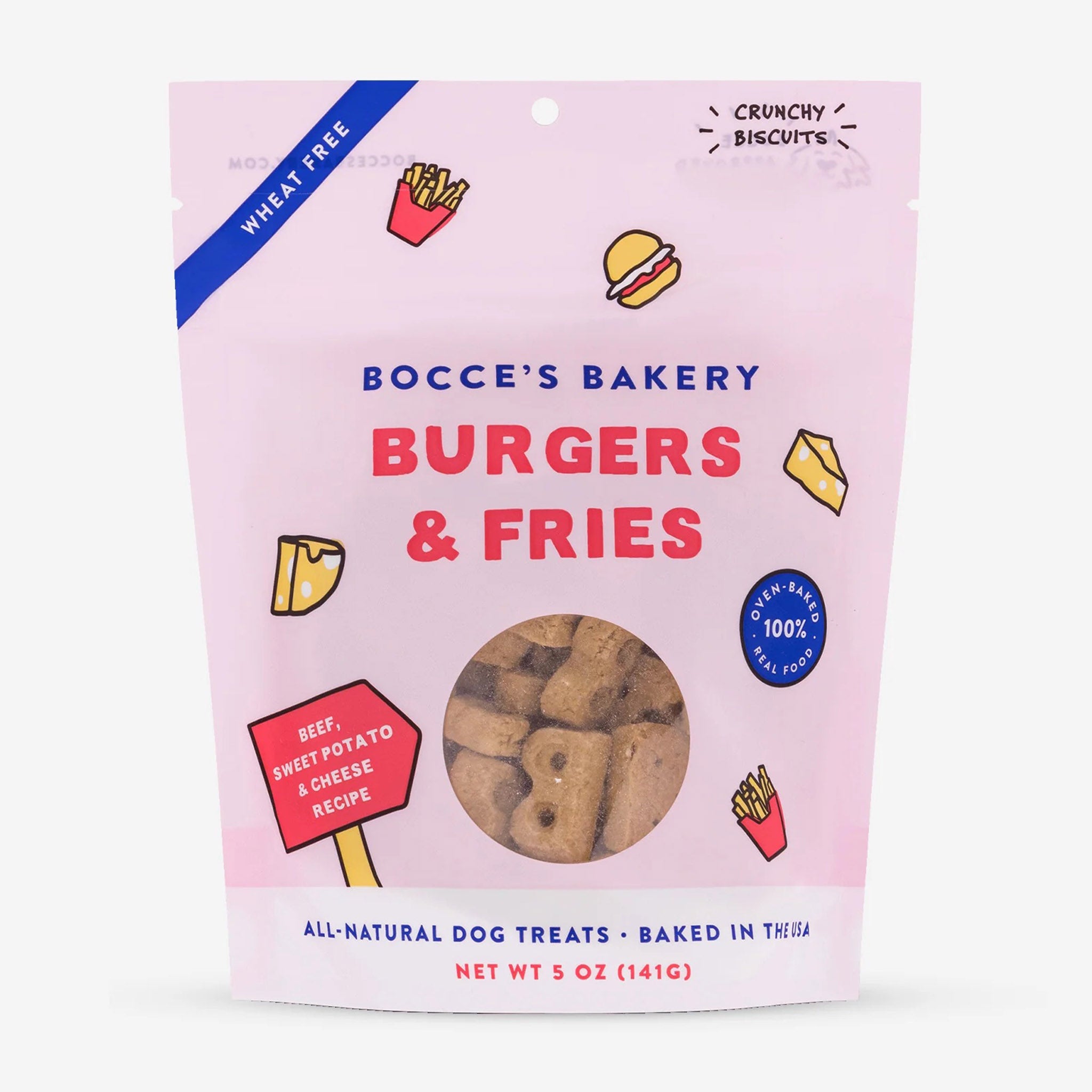This image showcases a close-up of a light pink package of dog treats called "Burgers and Fries" from Bocce's Bakery. The top left corner features a blue diagonal banner with "Wheat Free" text and illustrations of french fries and a hamburger. In the top right corner, the package indicates "Crunchy Biscuits." Central to the design, the brand name "Bocce's Bakery" is displayed in blue font, with "Burgers and Fries" in red font below it, flanked by images of cheese wedges. There is a translucent window in the middle of the package, revealing that the brown, crunchy biscuits inside are shaped like bees. Additional details include a red arrow in the bottom left corner stating "Beef, Sweet Potato, and Cheese Recipe," and text in blue and red fonts at the very bottom declaring the treats as "All Natural Dog Treats Baked in the USA," with a net weight of 5 ounces (141 grams). The overall background of the packaging design is white, emphasizing the vibrant colors and detailed graphics.